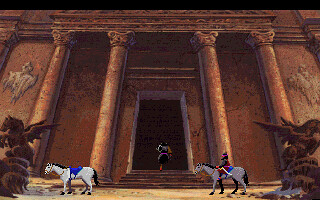The image features a tall, stately building reminiscent of colonial-era architecture, characterized by its brown facade. Dominating the entrance is a grand front door at the top of a flight of steps, where an individual is seen poised to ascend. Flanking the entrance, there are several statues. To the left, a striking statue of a horse rearing on its hind legs, with expansive wings extending from its back, captures attention with its intricate detail. In the foreground, two white horses are present. The first horse stands alone, adorned with a blue saddle and sporting a black tail. Behind it, another white horse similarly saddled in blue carries a rider, conjuring a scene of historic elegance and charm.